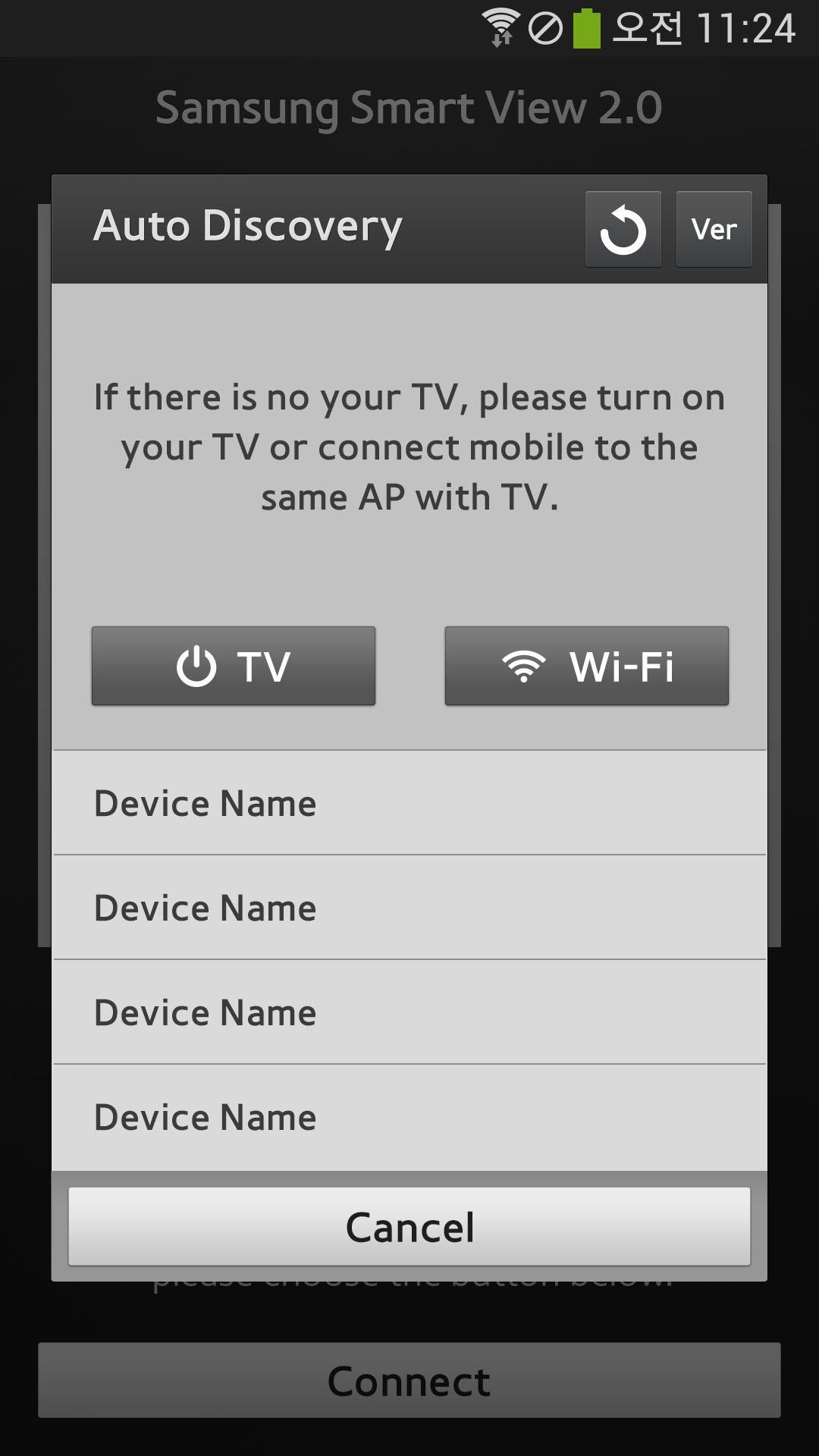The screenshot captures a phone interface connected to a Samsung Smart TV, currently encountering an error during channel discovery. At the very top, the phone's status bar displays the time, battery level, and signal strength icons, alongside some Korean text, suggesting the user's locale. Below this, the interface is titled "Samsung SmartView 2.0".

A prominent pop-up window for the auto discovery feature dominates the screen, offering "Refresh" and "Version" buttons in the top right corner. The error message within the pop-up reads, "There is no your TV. Please turn on your TV or connect mobile to the same AP with TV." Below this message, options for "TV" and "Wi-Fi" are presented, followed by a list comprising four rows of device names.

At the bottom of the pop-up, a "Cancel" button can be seen, just above which a "Connect" button is partially visible, indicating it belongs to the underlying interface rather than the pop-up window itself.